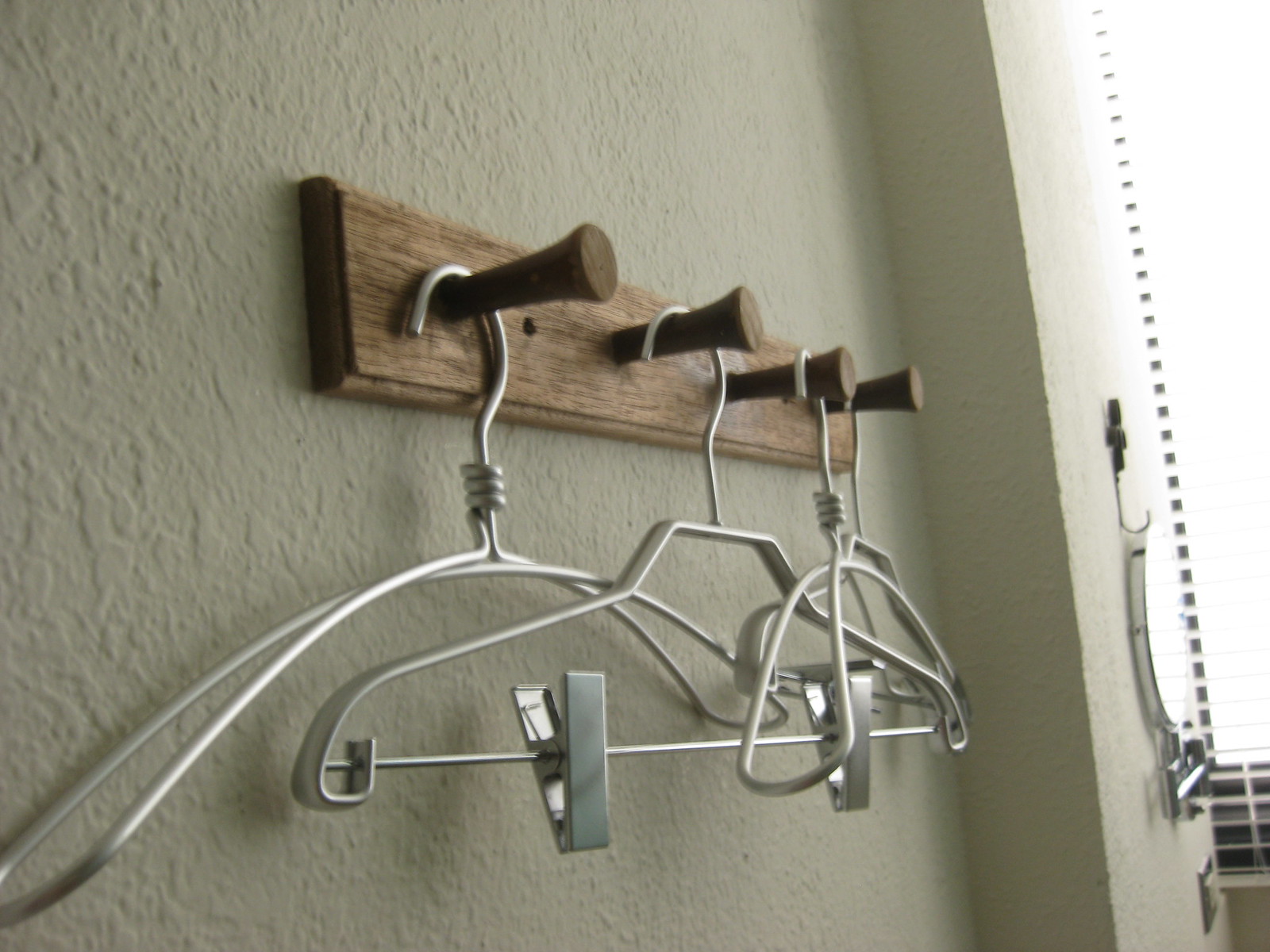The photograph depicts a close-up view of a light-colored wall, which appears to be either light gray or white plaster with a textured finish. Prominently featured on this wall is a rectangular wooden rack equipped with four wooden pegs. Each peg has a metal clothes hanger hanging from it. These metallic hangers are silver in color and vary in design; one of them specifically features additional clips at the bottom. To the very right edge of the image, a glass section is visible, but it's unclear whether it functions as a window or a mirror. Adjacent to this glass section, a black clip or metal hook is mounted on the wall, from which hangs a metallic tool or device, though its exact nature is indistinguishable due to the distance. The scene is bathed in soft, natural light, possibly from an unseen window casting a gentle glow over the arrangement.